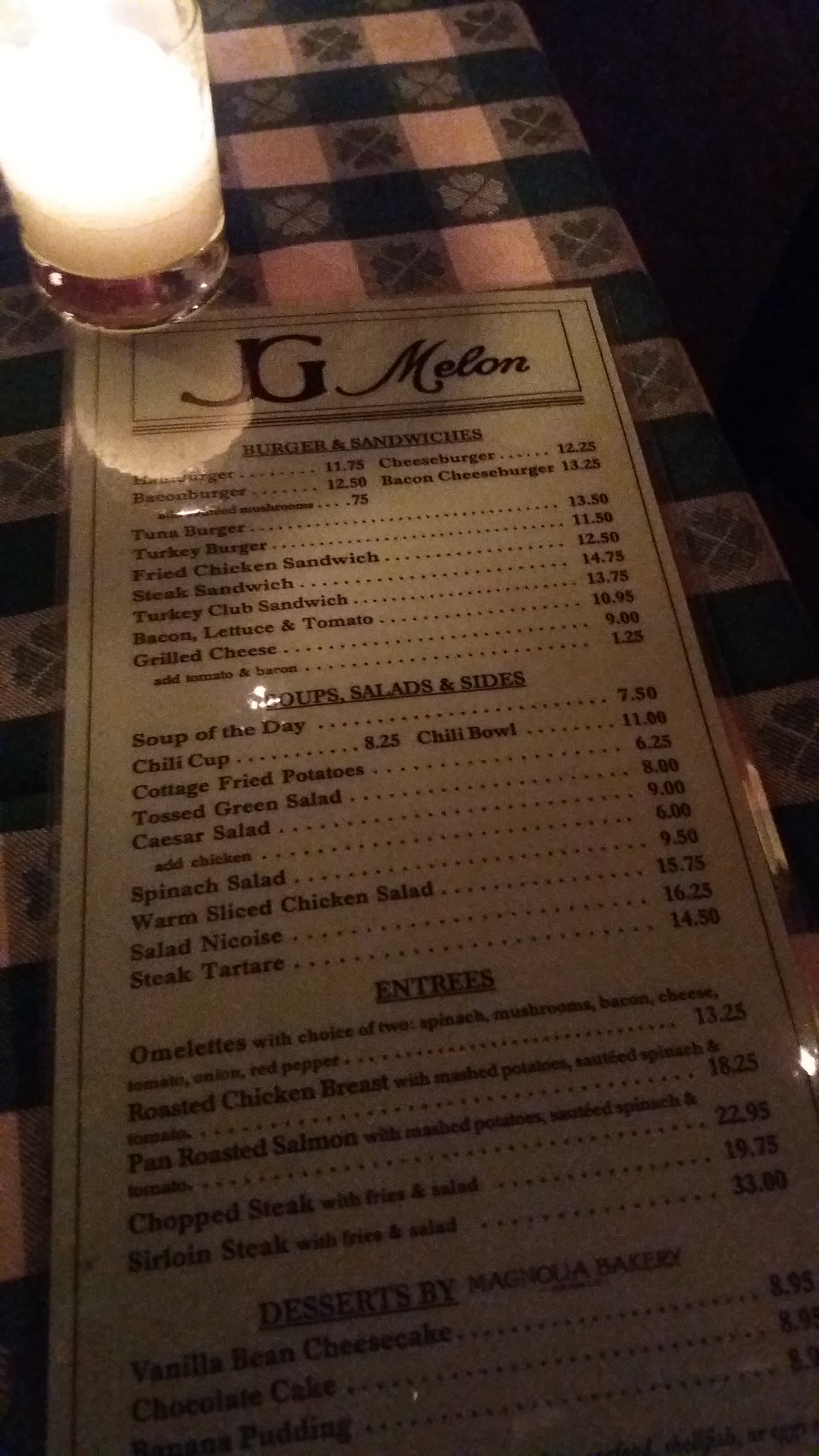In the upper left-hand corner of the image, there's a candle serving as a light source. The candle is housed in a clear glass container, with the base of the container also being transparent. The candle itself appears to be white, casting a gentle, white light. 

The background features a tablecloth with a pattern of colorful squares, including shades of gray, green, and white. Some of the green and gray squares are adorned with shamrock designs. The tablecloth suggests a festive or themed setting, although the exact shape of the table—whether rectangular or square—cannot be determined due to the zoomed-in perspective of the image.

In the center of the image is a menu. The menu is rectangular and seems to be an off-white color, possibly influenced by the lighting. The top of the menu displays the name "JG Melon." Below the title, the menu is divided into sections: "Burgers and Sandwiches," "Soups, Salads, and Sides," and "Entrees." At the bottom, the menu features a section titled "Dessert by Magnolia Bakery."

The menu items listed in the "Burgers and Sandwiches" section include:

- Bacon Burger for $12.50
- Cheeseburger for $12.25
- Bacon Cheeseburger for $13.25
- Tuna Burger for $13.50
- Turkey Burger for $11.50
- Fried Chicken Sandwich for $12.50
- Steak Sandwich for $14.75
- Turkey Club Sandwich for $13.75
- Bacon, Lettuce, and Tomato for $10.95
- Grilled Cheese for $9.00 (with an option to add tomato and bacon for $1.25)

This detailed description captures the essence of the image, highlighting the candle's ambiance, the festive tablecloth, and the detailed offerings of the menu from JG Melon.